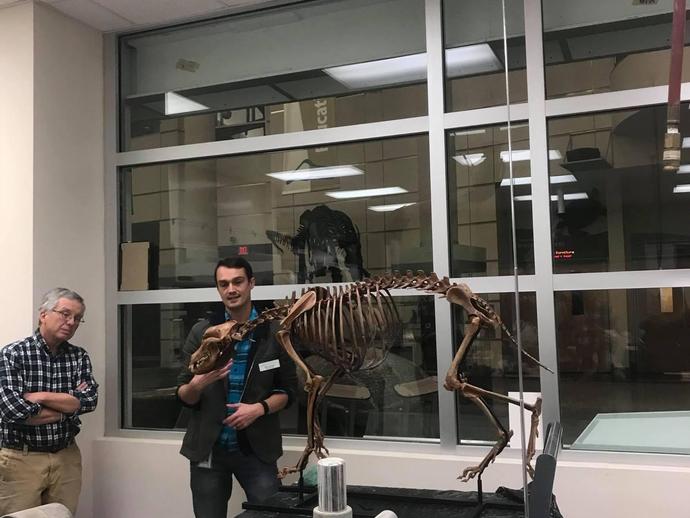In an exhibit room, possibly part of a museum or research facility, two men are engrossed in examining a fossilized skeletal creature of a four-legged animal, displayed on a black stand. The skeleton, which has a copper or dark brown hue, features a dog-like head, large teeth, and four paws, with an arched back and unique feet. The animal appears to be caught mid-stride, positioned as if walking towards the left of the image, held up by supporting pins.

The backdrop is a wall adorned with giant windows divided into nine sections by silver bars, showing reflections of the illuminated interior against the likely dark exterior. In the distance, behind the windows, faint outlines of additional exhibit items, walls, doors, and signs are visible.

The two men studying the skeleton are Caucasian. The one on the left, older with gray hair and glasses, wears a checkered black and white button-up shirt tucked into tan slacks and stands with his arms folded. To his right is a taller, younger man with dark hair, dressed in a black jacket over a blue and white shirt and jeans, who appears to be indicating aspects of the skeleton with his hand. A white name tag is pinned to the left side of his jacket. The detailed setting and attire of both men suggest a scholarly or curatorial context as they engage with the prehistoric exhibit.